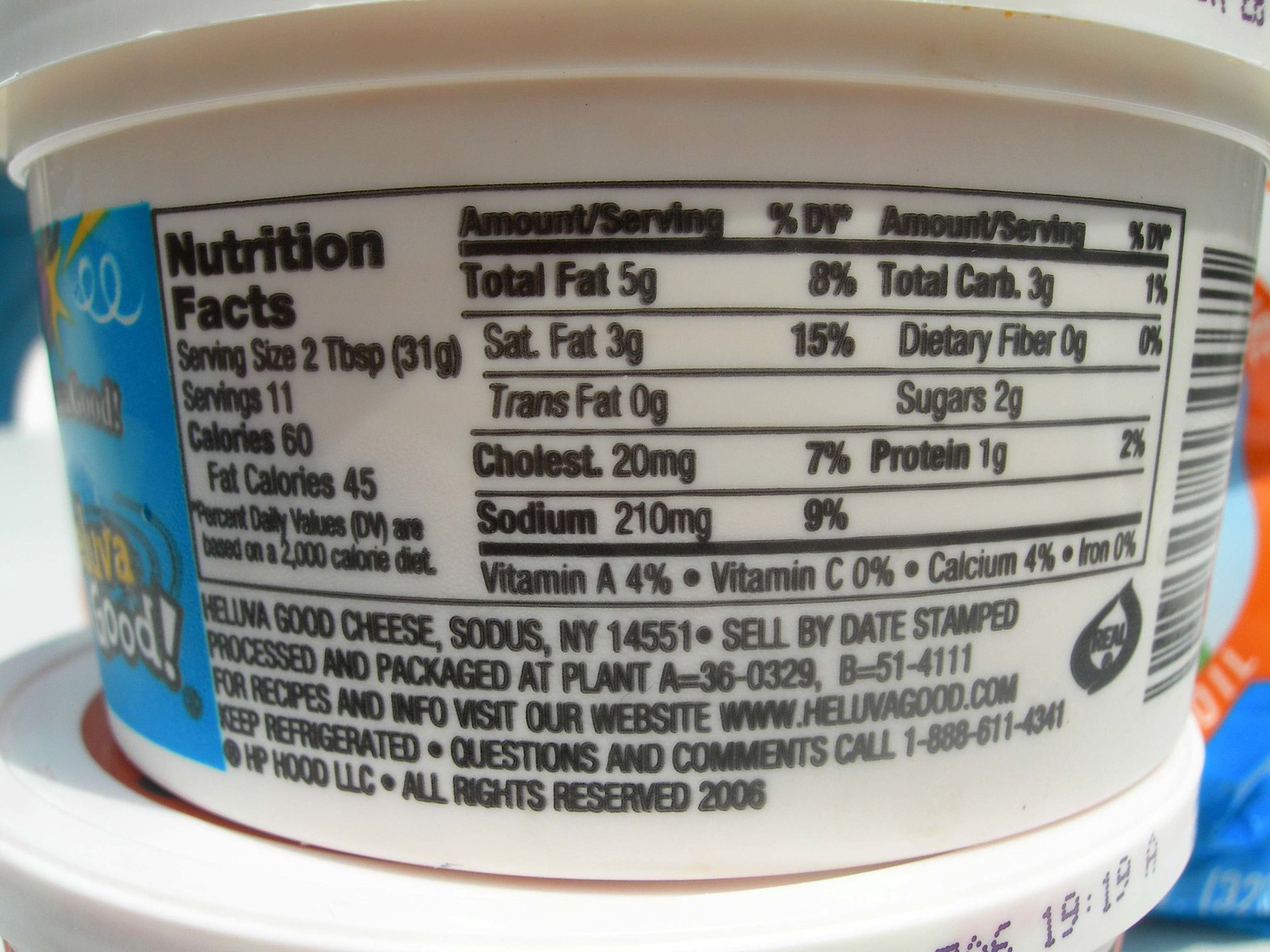The image showcases a white plastic tub containing a dairy product, presumably from the brand "Heluva Good!". Partially visible on the right side of the front label, the tub prominently features a blue background with bold yellow and white text spelling "Heluva Good!". Adjacent to this, the nutritional information panel is detailed, documenting key dietary information, including "Nutrition Facts," a serving size of "2 Tablespoons," a total of "11 servings," "60 Calories," and "45 Fat Calories," along with other percentage daily values based on a 2000 calorie diet. Beneath this panel, smaller text outlines the ingredients and additional packaging information, while a distinct black barcode resides to the right. The tub is positioned atop another identical tub, suggesting a stacked arrangement.